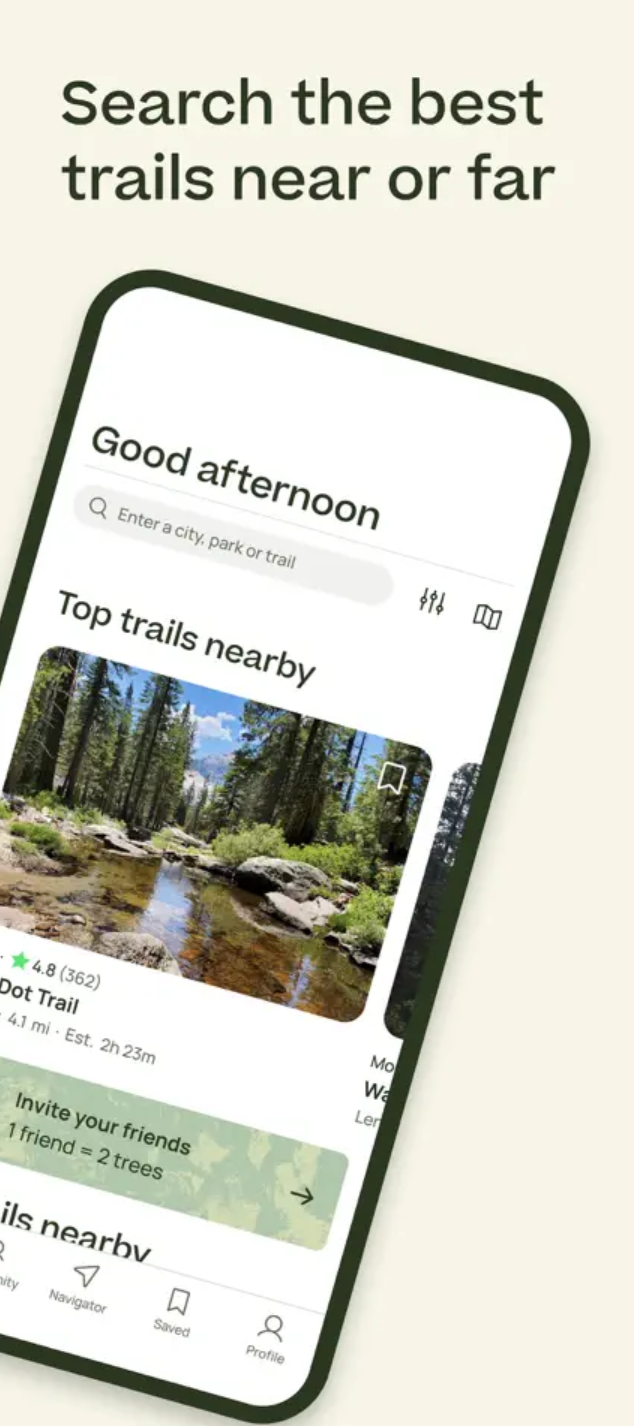The image features a light, off-white background that extends uniformly from left to right and top to bottom. At the top of the image, in bold black font, the text reads "Search the best trails, narrow or far." Positioned below this text is a close-up photo of a smartphone, slightly angled to the right, with its bottom left corner cropped out of the frame. The smartphone has a sleek black border and displays a user interface. At the top of the screen, a spacious white area hosts the greeting "Good Afternoon" in black, left-justified font. Directly beneath the greeting is a search bar that prompts users to "Enter a city, park or trail." Following the search bar, the text "Top Trails Nearby" is presented, accompanied by an image depicting the end of a body of water surrounded by rocks. In the background of this image, a dense, wooded area can be seen, adding a natural, serene element to the visual composition.